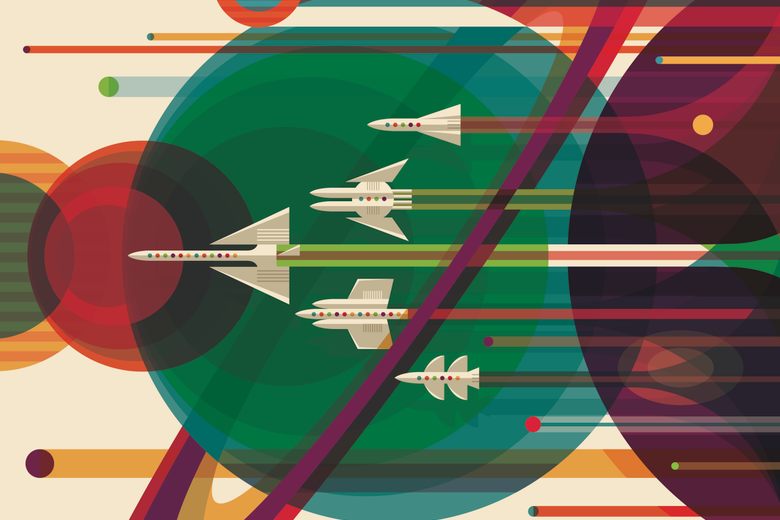The abstract image features a cream-colored background adorned with a series of overlapping circles, planes, and vibrant horizontal lines. Dominating the center is a pronounced blue circle housing additional green circles within it. To its left, there's a red circle, and farther to the edges, one can observe orange and green circles, interspersed with smaller shapes in varied hues of reddish, greenish, purplish, and brownish tones. 

Extending towards the left from the right-hand side of the image are multiple solid-colored horizontal lines in shades of orange, red, and green. These lines suggest motion as they trail behind what appears to be five stylized, sci-fi spacecraft. These spacecraft, rendered in a grayish-white color, exhibit a variety of intricate designs - one with a conventional appearance, another with dual heads, followed by one with triangle-shaped wings and an extended fuselage, another featuring three fuselages, and a final one resembling a standard spacecraft but with additional wings.

The planes align in a formation that brings to mind a swan in flight, their solid streaks extending across the image, simulating vapor trails. Noteworthy is the depiction's transparency, allowing for the superimposition of elements such as circles through other circles, creating a layered visual effect. The overall composition is meticulous, offering a blend of sharpness and semi-transparency, adding depth to the graphic design.